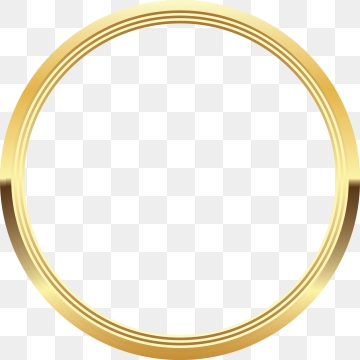An intricately designed gold ring, depicted in a 2D animation style, dominates the image against a backdrop of grey and white checkers, typical of transparent backgrounds in clipart. The ring's circular form is hollow at the center, allowing the checkered pattern to fill most of the screen around it. The top half of the ring gleams brightly, suggesting an overhead light source, while the bottom half features a darker shade of gold or bronze to convey a shadow effect, enhancing its three-dimensional appearance. Three concentric lines run along the interior of the ring, adding depth and a layered texture. The lighter lines within the ring contrast with its golden exterior, creating a sense of intricacy and realism, even though the entire depiction is unmistakably rendered in a 2D format.